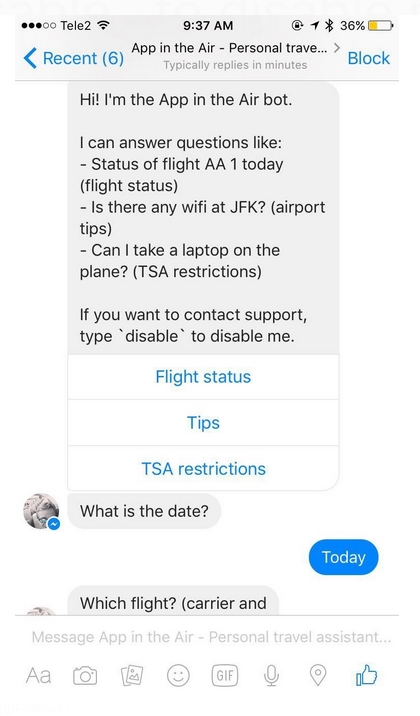The image is a screenshot of a customer service text exchange within a messaging system. At the top of the screenshot, there is a header that reads, "App in the Air - Personal Travel," followed by an incomplete phrase and a note indicating that the service "typically replies in minutes." 

The initial message in the exchange is from the automated bot named "App in the Air Bot." The bot introduces itself and outlines its capabilities by stating, "Hi, I'm the App in the Air Bot. I can answer questions like the status of flight AA1 today (flight status), if there is Wi-Fi at JFK (airport tips), and if you can take a laptop on the plane (TSA restrictions)." The bot also provides instructions on how to contact human support by typing "disable" to turn off the automated system. There are interactive buttons available for users to click on, labeled "Flight Status," "Tips," and "TSA Restrictions."

The conversation continues with a message asking, "What is the date?" The sender, located on the right side of the screen, responds with "Today." The last visible message is from the bot, asking, "Which flight carrier and..." with the rest of the message cut off.

This detailed screenshot captures the dynamic interaction between a user and a customer service bot designed to assist with travel-related inquiries.